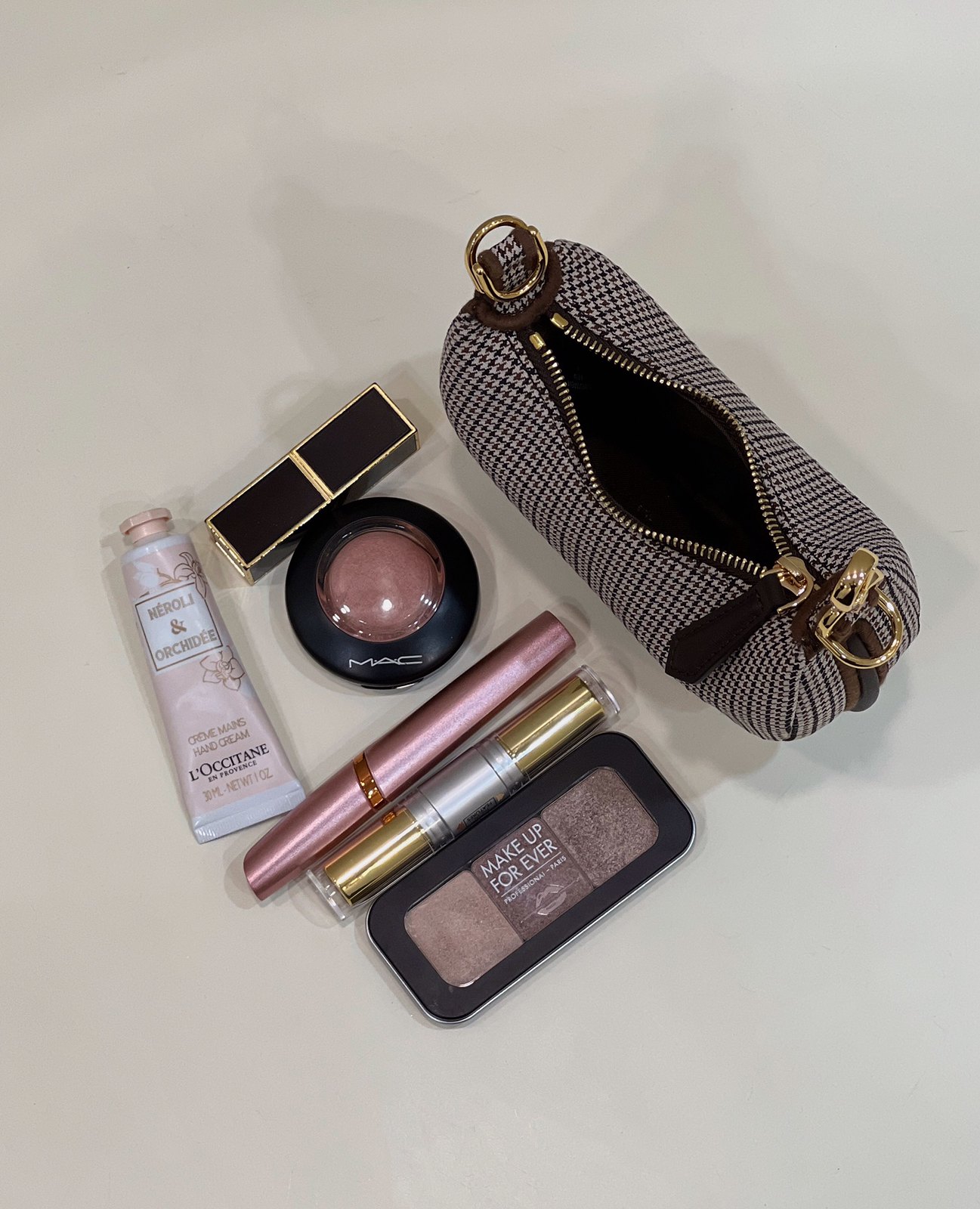In the upper right corner of the image, there is a makeup pouch or purse adorned with a tightly woven grid pattern featuring black and grey hues. The pouch has an open zipper running across the top, showcasing gold-toned teeth. The zipper's black handle angles down toward the bottom left. The purse also features gold-colored rings positioned at the upper left and bottom right corners. Additionally, a copper-colored clasp is visible on the bottom right side.

Spread out to the bottom left of the purse are various items. At the top of this arrangement, a bronze-toned rectangular box with a row of black rectangular accents in the center and gold detailing catches the eye. Below this is a black circular object with a noticeable bulge of purple color at its center. Further down is a long, cylindrical pink device accented with a gold circle around it. Adjacent to this item is another long cylinder, characterized by gold ends and a silver middle section.

Continuing the array, a long rectangular item with black rounded edges bears the inscription "Make Up Forever." This item has two color sections beneath the text — one is a solid purple, while the other features a blend of purple and gray hues. 

To the left of these items, there is a squeeze bottle adorned with a central white square label, which contains hard-to-decipher lettering. However, the word "L'OCCITANE" is clear near the bottom of the label. This bottle is further distinguished by its pink cap.